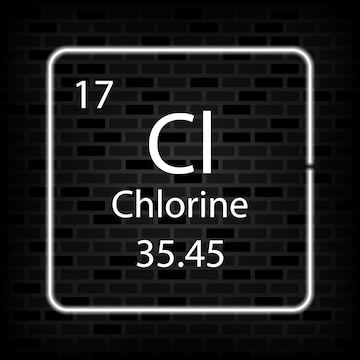The image features a detailed depiction of a neon-like white square, slightly rounded at the corners, superimposed against a predominantly black background with a subtle brick pattern that varies in shades of black, gray, and light gray, gradually fading to pure black towards the edges. Inside the white outlined square, the number "17" is prominently displayed in the upper left corner. At the center of the square, the chemical symbol for chlorine, "Cl" (with a capital 'C' and lowercase 'l'), is boldly featured. Directly below this symbol is the word "chlorine" written out in white letters, followed by its atomic weight "35.45." Notably, there is a small gap on the right side of the square’s otherwise continuous outline, creating a slight break in the neon-like border.